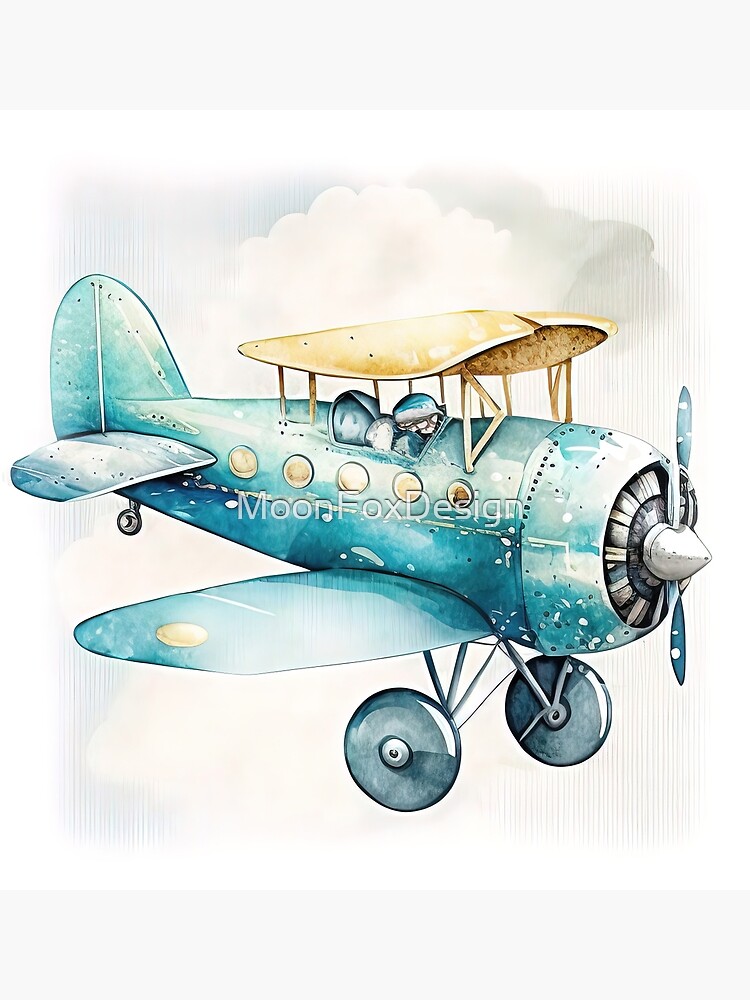The whimsical digital artwork showcases a small, vintage propeller airplane in mid-flight, resembling a classic biplane. The aircraft is primarily a teal blue color with white highlights, featuring a distinct upper wing that is a yellow-brown hue. This upper wing is connected to the fuselage with supporting struts but does not extend as wide as the lower wing beneath the pilot. 

The open cockpit reveals a pilot wearing goggles and a protective helmet, seated without a glass canopy, just an awning, indicating the plane may not fly at high altitudes. The front of the airplane is equipped with a stationary, two-blade propeller, suggesting movement despite its static depiction.

The airplane's fuselage is adorned with yellow circles, similar to portholes, although they seem decorative as there's only room for the pilot. A similar yellow circle marks the tip of the right wing. The landing gear consists of two large, permanently fixed front wheels and a smaller rear wheel. The artwork is set against an off-white background with faint cloud shapes, adding to the whimsical, hand-drawn or painted appearance of the scene. Subtly, a watermark reads "Moon Fox Design," further lending an artistic touch to the piece.